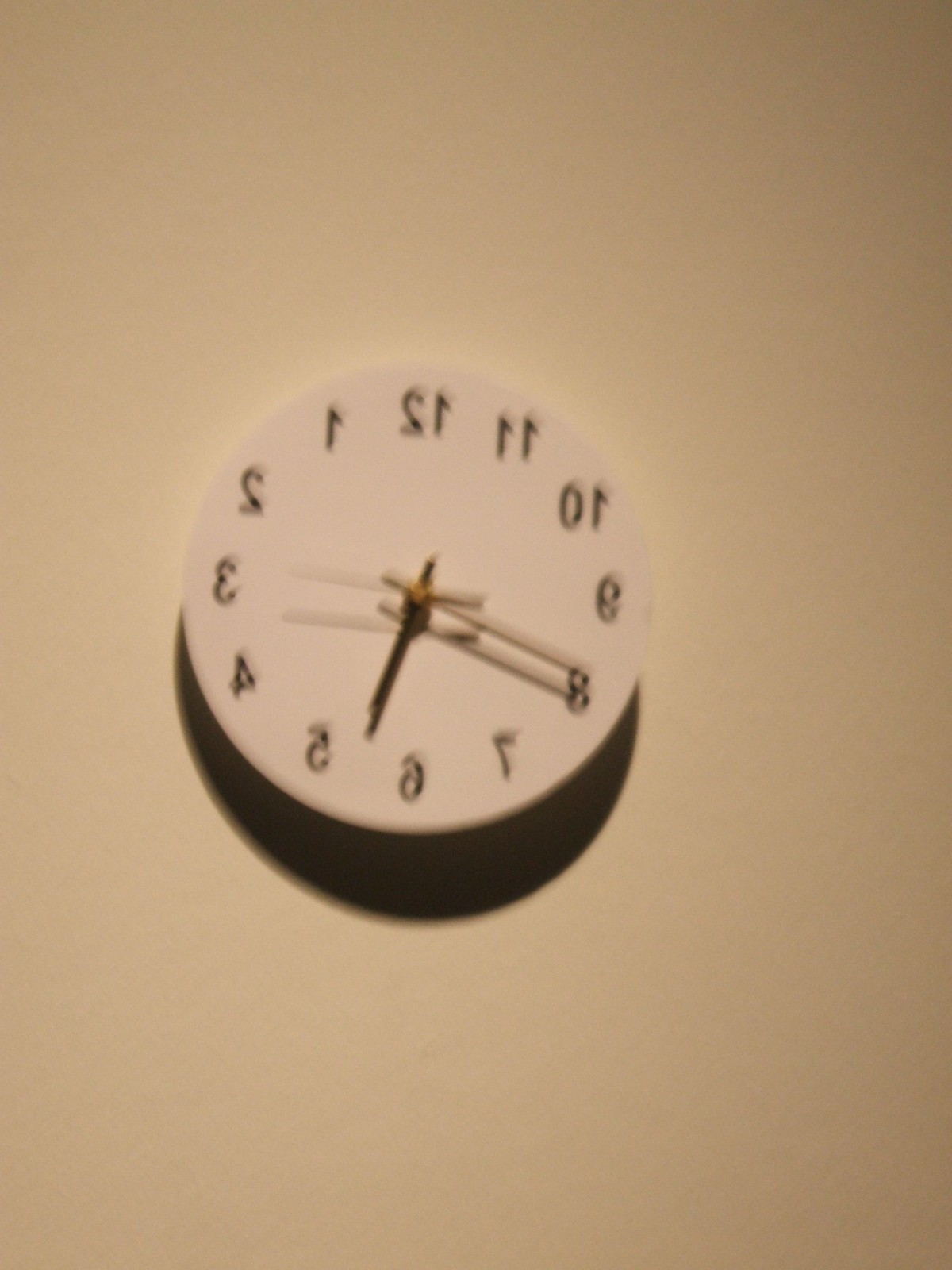The image depicts a wall clock that appears entirely white or soft cream in color, with no outer rim or border. The clock face is round, and it casts a shadow on the bottom creating a half-circle effect. Intriguingly, the numbers are oriented in a backward, counterclockwise direction, giving the impression that the image was captured through a mirror. The black hour and minute hands are almost identical in length, while a longer, red second hand runs briskly around the clock. The time displayed is approximately 5:40, with the hour hand situated between the 5 and 6, and the minute hand pointing at the 8. Black numbers from 1 to 6 appear on the left side, while 7 to 12 are positioned on the right side of the clock face.